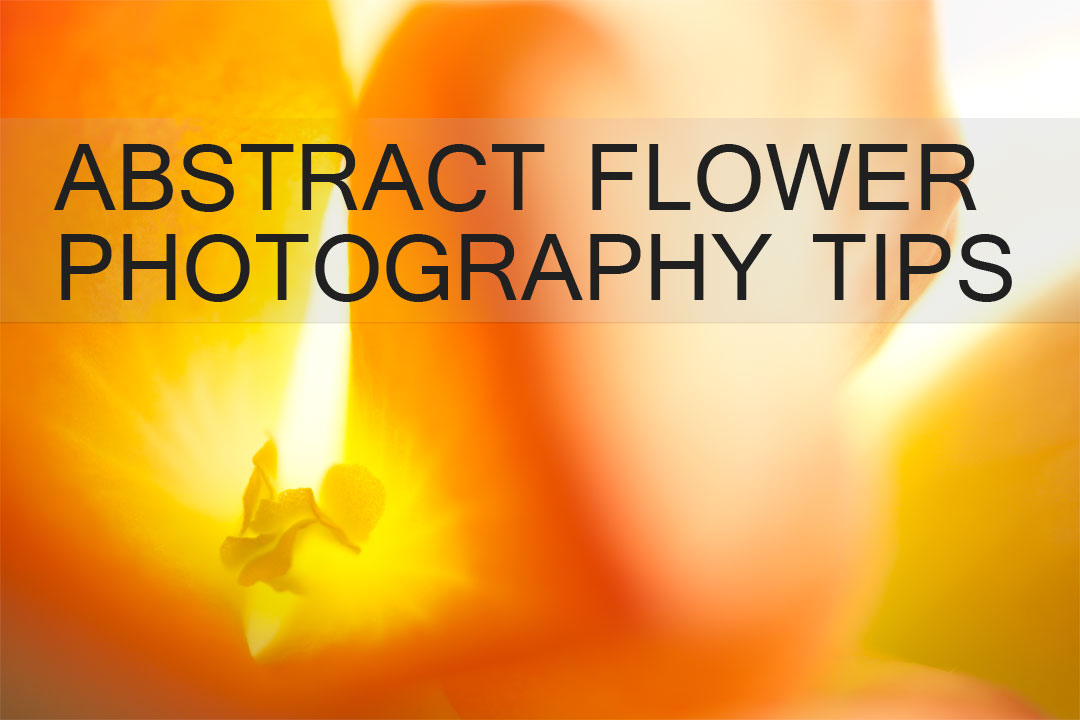The image features an abstract photograph of an orange flower with a yellow, sun-like center, enveloped by swirling petals. The composition creates a blurry, dreamlike effect with a blend of colors that graduate from yellow at the core to deeper shades of orange, interspersed with lighter hues of pink and white. The petals, which appear large and crinkled, extend outwards, giving the impression of rays emanating from the center. The photo's upper middle section is overlaid with a semi-transparent, frosted banner containing black text that reads "Abstract Flower Photography Tips." The background has hints of blue and additional yellow elements, contributing to the overall ethereal quality of the image.